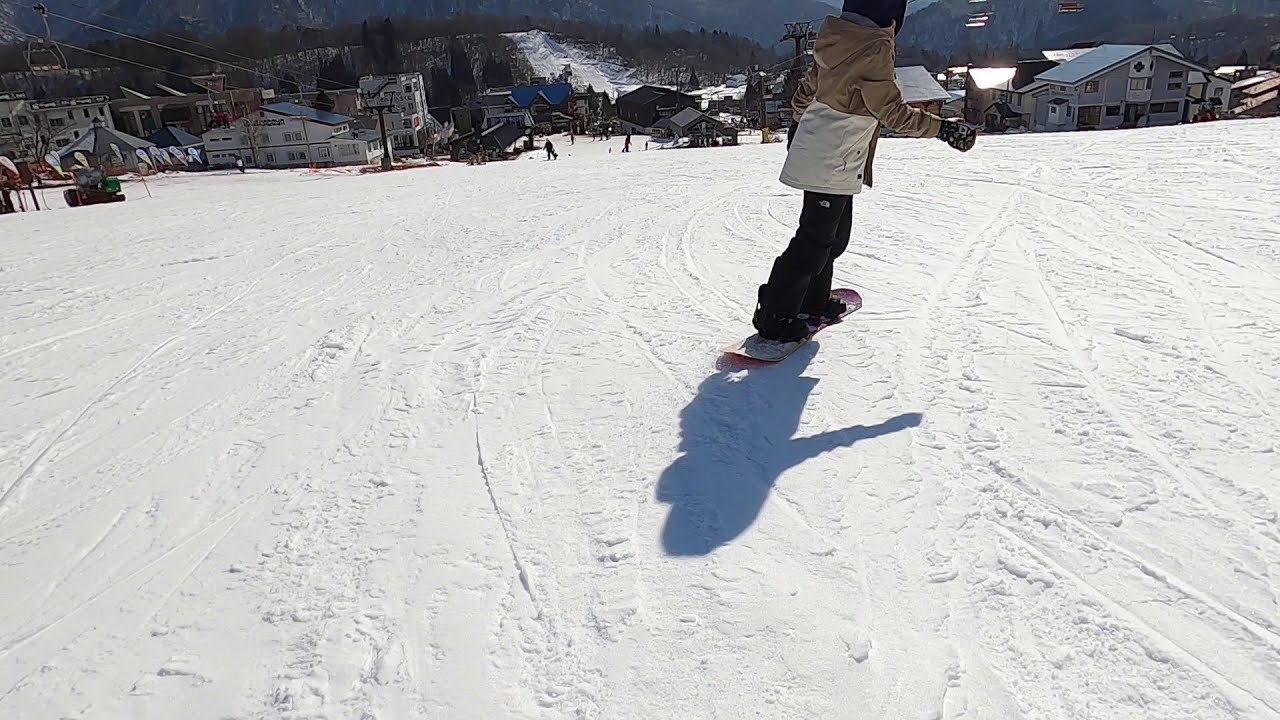This detailed color photograph, likely a freeze-frame from a GoPro video mounted on a snowboarder's helmet, captures a snowboarder in motion on a snow-covered slope in a wintertime town. The snowboarder, dressed in a tan-and-white jacket with a hood, black trousers, black gloves, and a black helmet, rides a red snowboard down the hill. The daylight scene is filled with tracks in the snow, left by previous skiers and snowboarders. To the left side of the image, a ski lift ascends, its wires stretching upward, with buildings and possibly ski lodges lining the area. In the background, a hill rises, dotted with leafless trees, and more individuals can be seen either skiing or walking. The snowboarder’s shadow is distinctly cast on the snow behind them, adding a dynamic element to this picturesque, realistic snapshot of a bustling ski resort area.